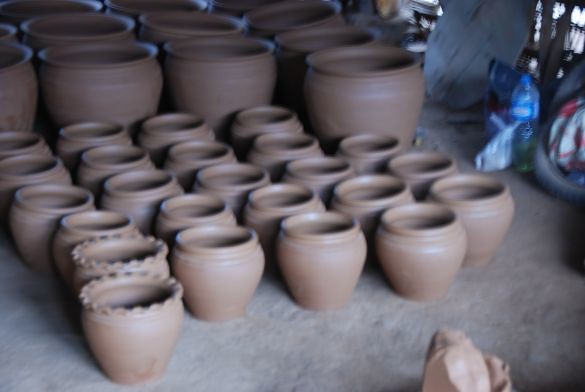In the photograph, there is an array of pottery bowls crafted from creamy-colored clay, neatly arranged on a light brown cement floor in what appears to be a workspace or garage. The foreground features rows of smaller bowls, each predominantly of the same size and simple round shape with a short, vertical lip. Among these, two distinctive bowls stand out due to their scalloped, serrated rims. These front rows consist of six bowls in the first column, followed by columns with five and three bowls respectively.

Behind this organized display of smaller pottery, there are approximately six to eight much larger pottery vessels, at least twice the size of the ones in front, extending into the background. Interspersed among the pottery, particularly on the right side of the image, are various items including a blue-capped water bottle with a blue sticker, a plastic bag, and assorted trash. A blue object of indeterminate purpose is also visible, adding a splash of color to the scene. A black tire can be spotted on the right side of the image, further indicating the utilitarian nature of the space. The consistent clay color, ranging from creamy to brownish tones, unifies the diverse assembly of pottery.